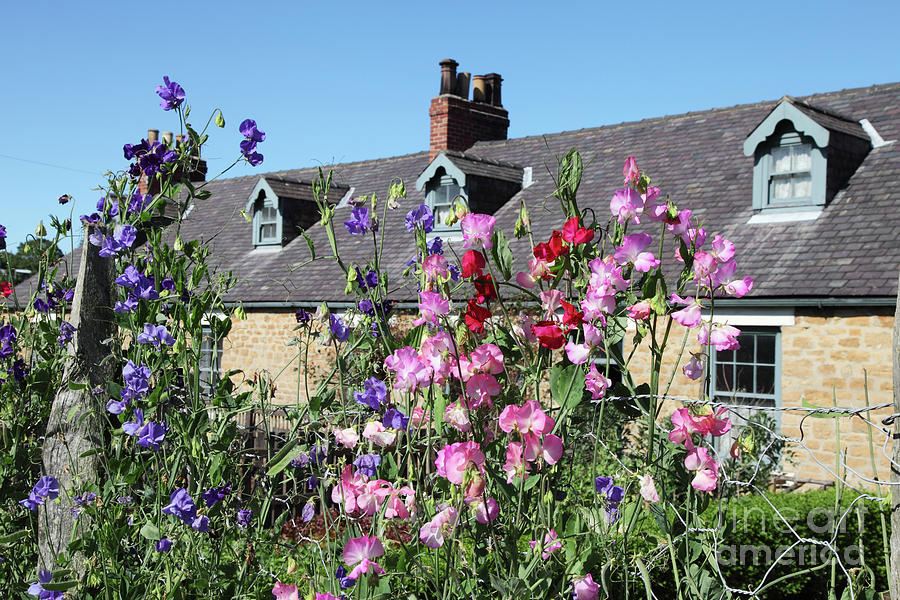A horizontal, color photograph captures a picturesque European stone house in the background, characterized by its expansive, yellow stone-like exterior, dark, prominent windows, and a central brick chimney. The slate roof and multiple gables add to its rustic charm. The house stretches across the entire frame, nestled under a pristine, clear blue sky. Dominating the foreground are vibrant, untamed flowers—pink, purple, and red blooms—set against long, green grass, lending a wild, natural beauty to the scene. The colorful flowers seem to frame the house, drawing attention away from its grand structure and celebrating the lively, natural growth that envelopes it.